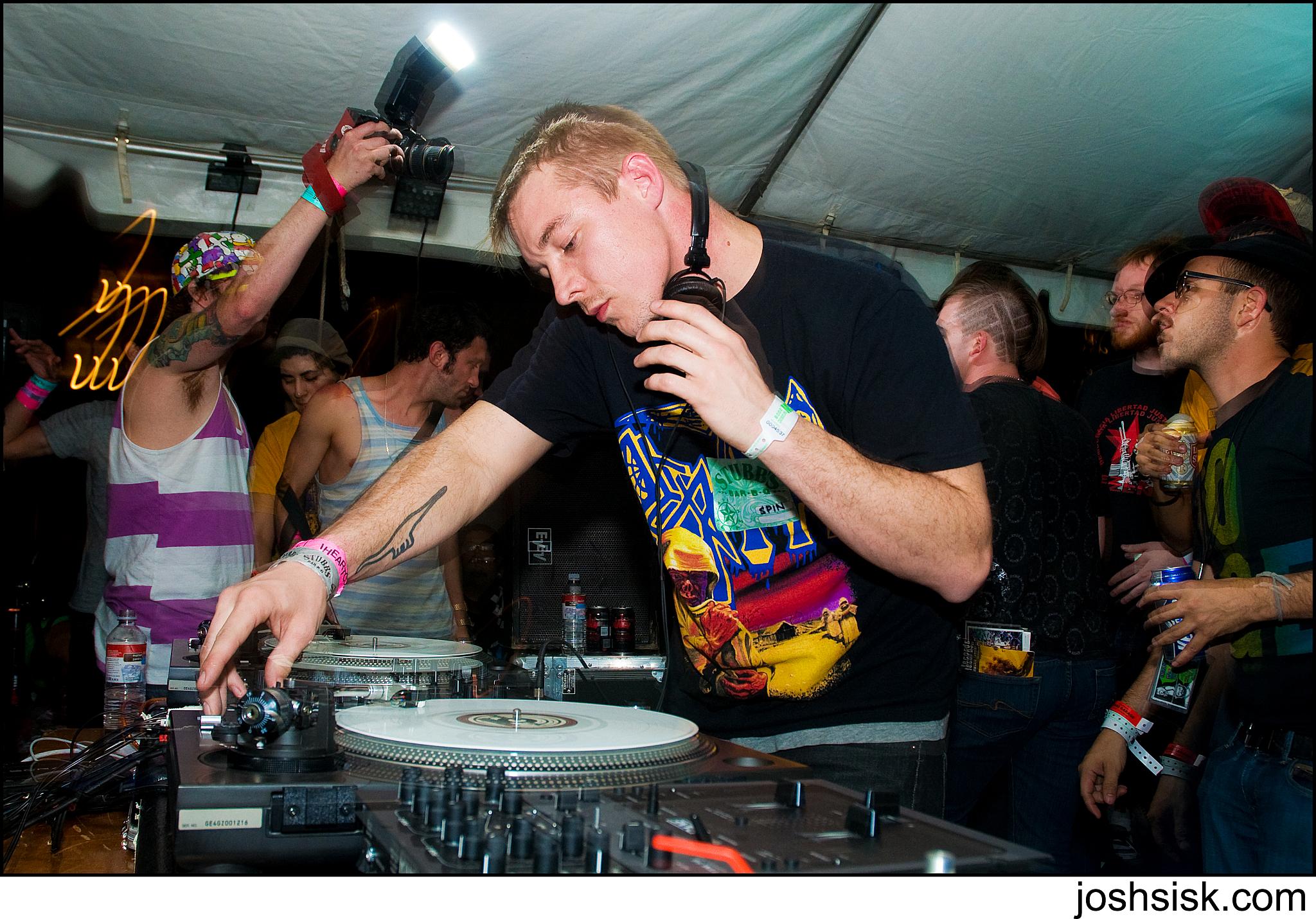The photograph measures approximately six inches wide and four inches tall, bordered by a thin black line. The photo credit "josh sisk dot com" appears in lowercase black print at the bottom right corner. Centered within the image is a young Caucasian man, likely in his late 20s to mid-30s, captured from the waist up as he leans over a turntable mixer, deeply engaged in crafting music. He has short blonde hair and wears a short-sleeved black shirt adorned with indistinct designs featuring blue and yellow elements. Around his neck rests a pair of over-the-ear headphones, which he grips with his left hand while his right hand manipulates the mixer. A tattoo of a dinosaur outline, possibly an Apatosaurus, is visible on his right forearm. 

Surrounding him is a lively crowd, blurred slightly to suggest motion and dancing. Notably, a man to the left is poised with a camera raised high, likely capturing the event. Above, the white underside of a tent is discernible, casting doubt whether the scene is indoors under a tent or outdoors at night under a tent. There's a hint of external view showing what appears to be a street sign, adding to the ambiance of an outdoor night event.